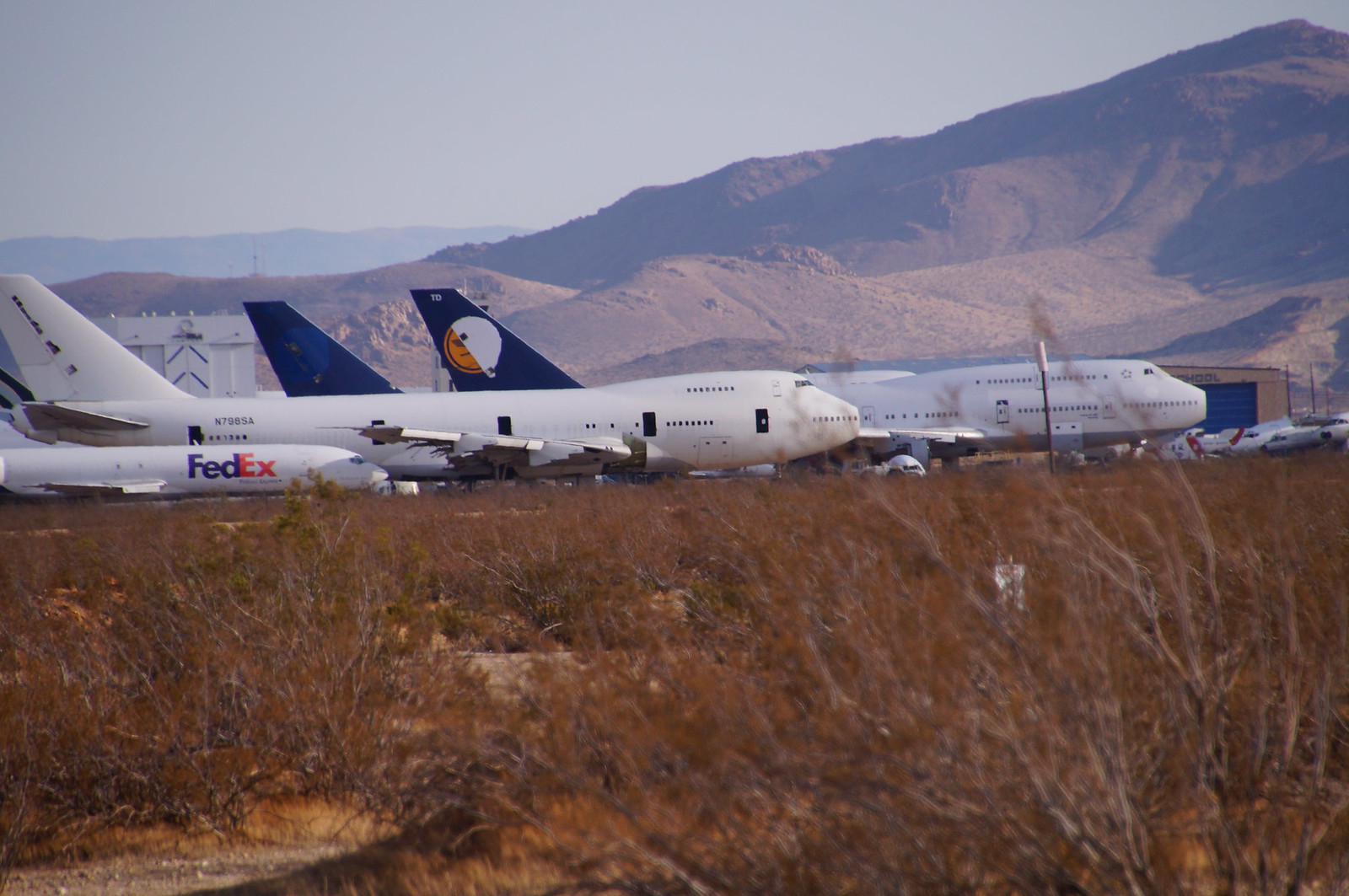The photograph captures a stark, deserted airport set in a barren, desert-like landscape. The foreground features scrubby, dried brown plants and patches of sand, which transition into a cluster of large airplanes grounded on an airstrip. Several of these planes, predominantly jumbo jets, are facing to the right. Notably, a smaller FedEx plane is prominently visible among them. The larger jets include models resembling 747s, with distinctive high bumps in the fronts. Two of these jets have blue tails, and one features a yellow and white logo in the center of its tail. Smaller vehicles and possibly smaller planes are faintly visible near the jets' noses.

In the background, there are two buildings: one small, low-slung hangar and a larger, ambiguous structure off to the left. Beyond the built environment, the landscape rises into rocky, barren hills covered with dried grass and brownish plant life. Further in the distance, additional hills and mountains fade into a gray, foreboding sky, completing the desolate scene. This combination of elements—desert flora, grounded planes, and remote mountains—suggests a storage or overflow area for aircraft, isolated in a sparse part of the desert.